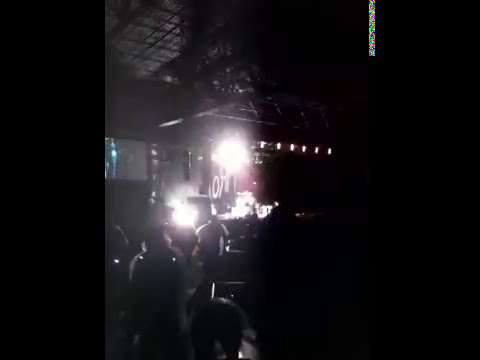In this mysterious and dimly lit photograph, the focal point is a vehicle positioned towards the center left, emitting a bright, illuminating light from its rear, which casts a glow on the surrounding area. Surrounding the vehicle, the image captures the backs of several people standing on the ground, though their features are indistinct due to the low light conditions. The overall ambiance of the image suggests it was taken indoors, possibly within a building, given the visible roof structure. The scene is bathed in shades of black, white, and gray, adding to its enigmatic aesthetic. On the top right, a vertical strip of colorful light contrasts with the darker hues, while two vertical black strips frame the left and right edges of the photograph, lending an additional sense of depth and framing. The image is so dim and blurred that specific details of objects or the exact nature of the scene are ambiguous, leaving much to the viewer's imagination.